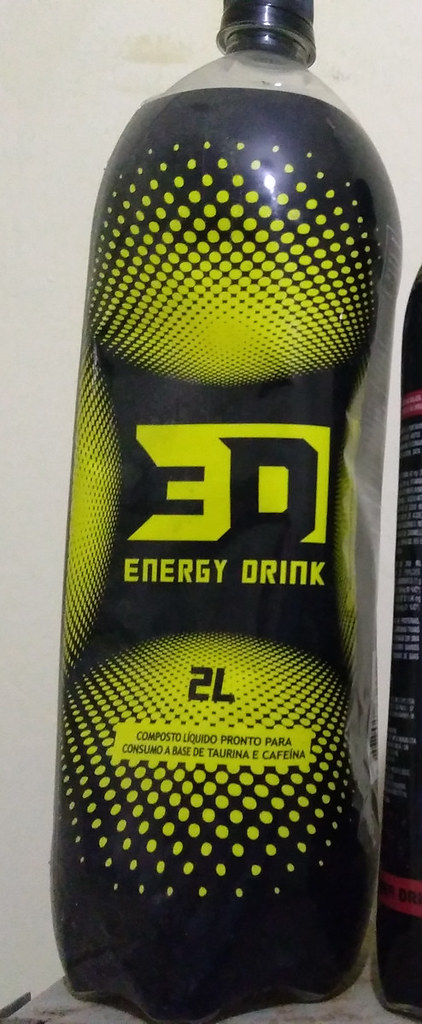A high-resolution image showcases a 2-liter bottle of an energy drink named "CD." The label commands attention with its predominantly black background adorned with sporadic yellow dots. Central to the label is a unique design element: a black square with inwardly curved edges, giving it a distinctive, modern appearance. Prominently displayed in the middle are bold block letters spelling "3D," with the numeral '3' in a striking yellow or light green hue, and the letter 'D' in classic black. Directly beneath this, the text "energy drink" is inscribed in vibrant green or light green, maintaining the energetic theme. At the very bottom of the label, the capacity is clearly marked as "2L." Adding a touch of bilingual detail, a green banner runs underneath this, featuring a Spanish phrase: "composto líquido pronto para consumo a base de taurina y cafeína," indicating that the liquid composition is ready for consumption and contains taurine and caffeine.